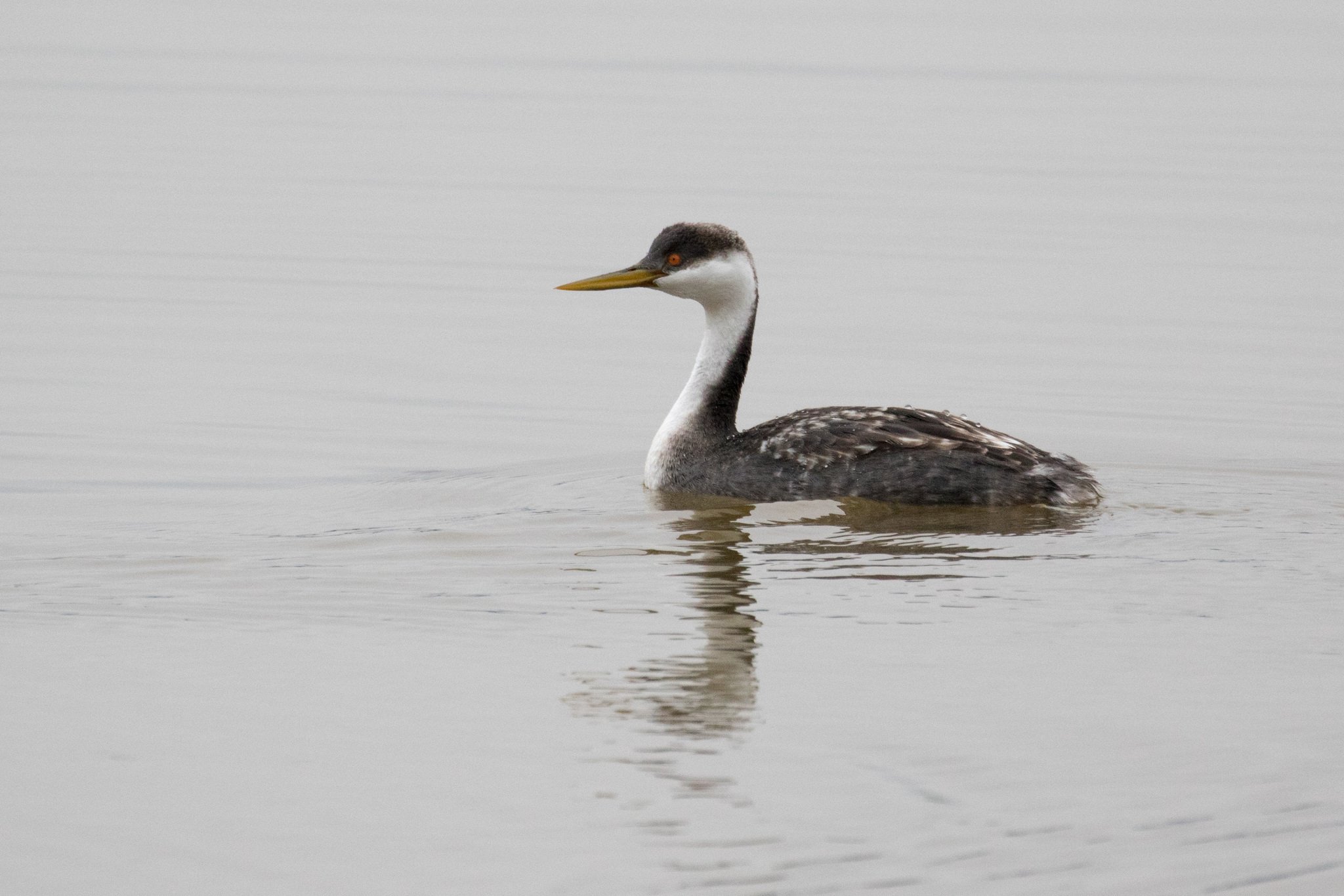A detailed nature photo showcases a duck swimming in a body of water, likely a lake or pond, under overcast skies. The water has a grayish-blue tone, suggesting it could be an overcast day. The duck, facing and moving to the left, disturbs the surface, creating subtle waves. This duck features a distinctive orange bill with a sharp point and striking reddish eyes. Its head has a gradient of colors: gray feathers cover the top, transitioning to white running down the neck and chest. The back of the head and top also have brown feathers that wrap around to the neck. The duck’s body is predominantly gray with brown, and it has tiny white specks on its wings that are tucked in. Given the absence of other ducks and the murky, brownish water, the setting appears solitary and tranquil. The lighting suggests it is daytime, but the lack of bright sunlight hints at an early morning, late evening, or overcast atmosphere.